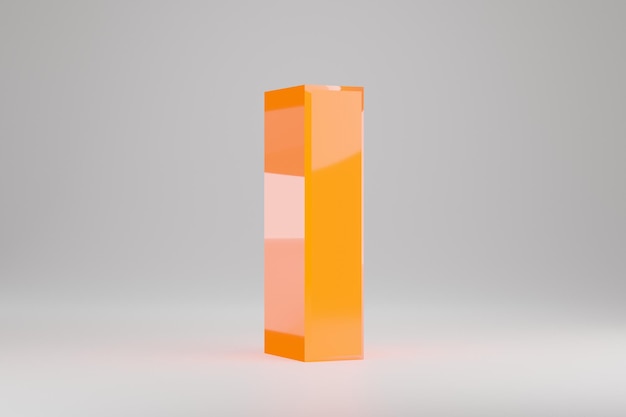The image features an animated, orange rectangular prism that stands prominently against a blurred gray background, which gradually transitions from a lighter gray at the bottom to a darker gray at the top. The prism has sharp corners and smooth surfaces, with two visible sides exhibiting different shades of orange. The front of the prism showcases a bold, vibrant orange, while the side transitions from a darker orange at the top to a lighter, almost whitish orange in the middle, before becoming dark again at the bottom, reminiscent of a sunset gradient. This reflective quality of the prism casts a soft, warm orange light onto the lighter gray floor beneath. The object appears to be three to four times taller than it is wide, emphasizing its verticality. The overall aesthetic suggests a basic 3D animation, possibly created using modeling software.